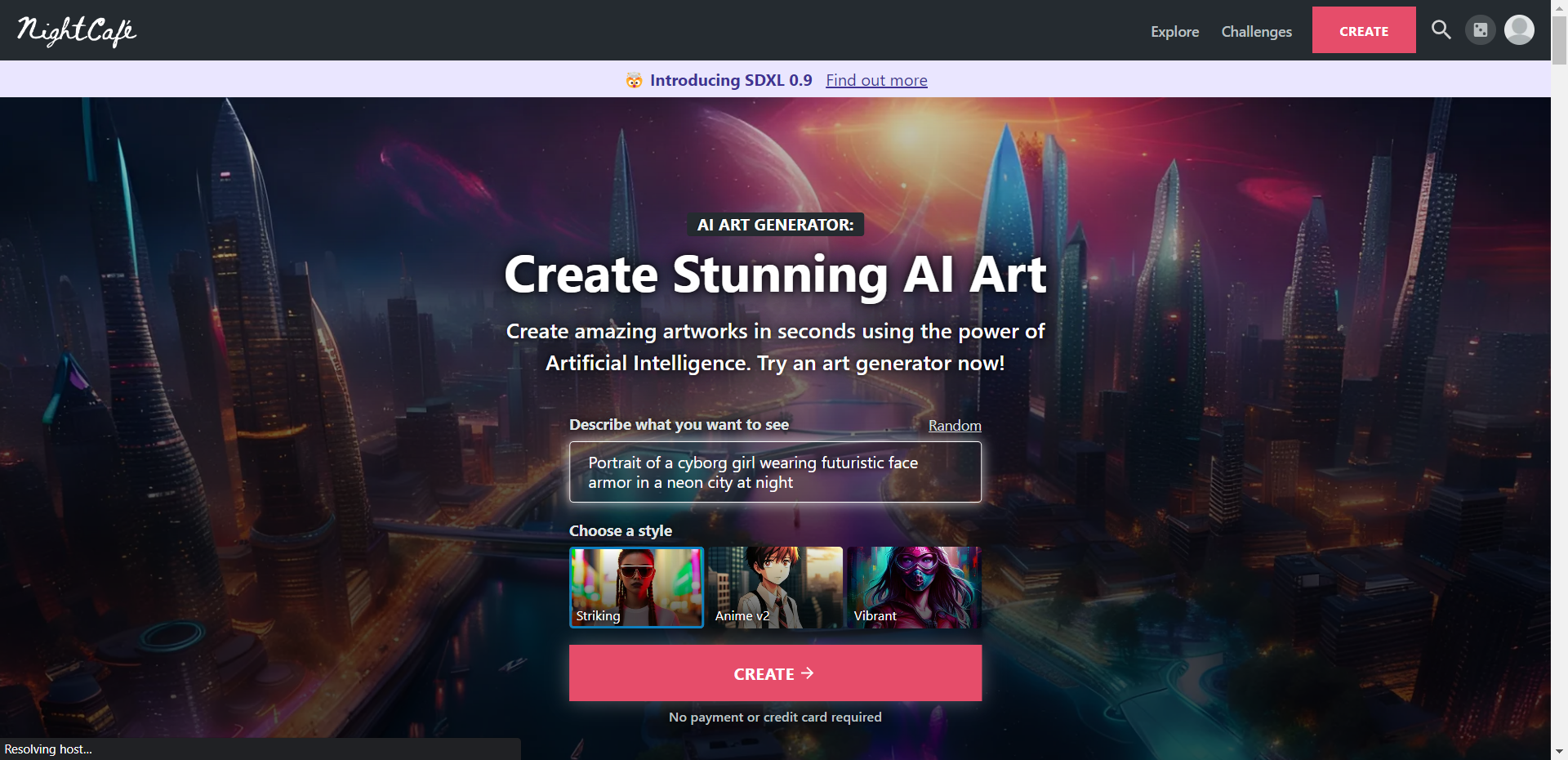The image depicts the Night Cafe website interface, showcasing its main features. At the top, there is a black header bar displaying the Night Cafe logo. Within this bar are various menu options: 'Explore,' 'Challenges,' and a prominent red 'Create' button. Additionally, there is a magnifying glass icon signifying a search function, followed by two circles—one with an unspecified symbol and the other with a generic user profile icon.

Below this, a light white bar spans the width of the page, prominently featuring an emoji and the text "Introducing SDXL 0.9" in all capital letters, accompanied by a "Find Out More" link. 

The main section of the homepage displays a captivating cover image with a black rectangular box that boldly announces "AI Art Generator" in white text. Beneath this, a tagline in white text reads, "Create Stunning AI Art." Further down, there's a descriptive sentence: "Create Amazing Artworks in Seconds, Using the Power of Artificial Intelligence. Try an Art Generator Now." 

Users are invited to describe their desired artworks in a designated text box, with an option to generate random art. They can also choose their preferred art style before clicking the 'Create' button, which is highlighted in red with a rightward-pointing arrow. This detailed layout emphasizes the website's focus on enabling users to create AI-generated art effortlessly.